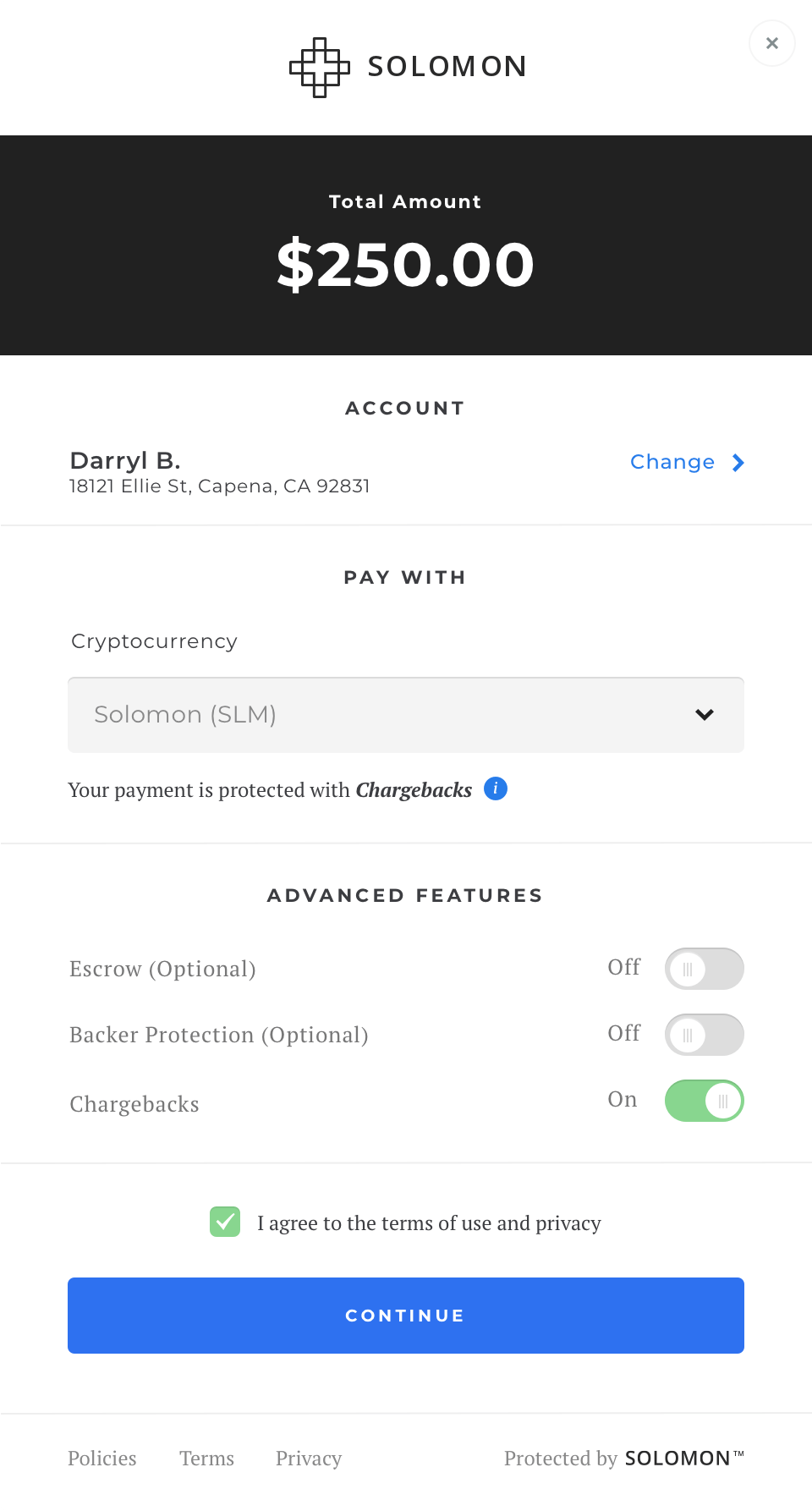Screenshot showing the Solomon cryptocurrency payment interface on a smartphone screen. The background is predominantly white. At the top center, "Solomon" is displayed in black text, to the left of which is a square emblem featuring a "T." 

Below the emblem, a black rectangle prominently displays the white text, "Total Amount: $250," with the "$250" in bold. Further down, the word "Account" is written in black text. To the left beneath it, the details read: "Daryl B., 18121 L.A. Street, Copenha, California 92831." Meanwhile, to the far right in blue text, the word "Change" is visible, accompanied by a right-pointing directional arrow.

The section titled "Pay With" is centered below this, written in black text. Underneath, to the left, the word "Cryptocurrency" is mentioned. A long, light gray rectangle follows, labeled "Solomon (S.L.M.)," which appears to be a drop-down menu to the right.

Beneath this, in black text, the phrase "Your Payment Is Protected With Chargebacks" is displayed. Below it, under "Advanced Features," two optional settings are listed: "Escrow (optional)" and "Backup Protection (optional)," both of which are set to "Off." The term "Chargebacks" is listed next, to the right of which is "On."

Below these options, a statement reads: "I agree to the terms of use and privacy," next to a green check-marked box. At the bottom of the screen, a blue rectangle with white text indicates the "Continue" button.